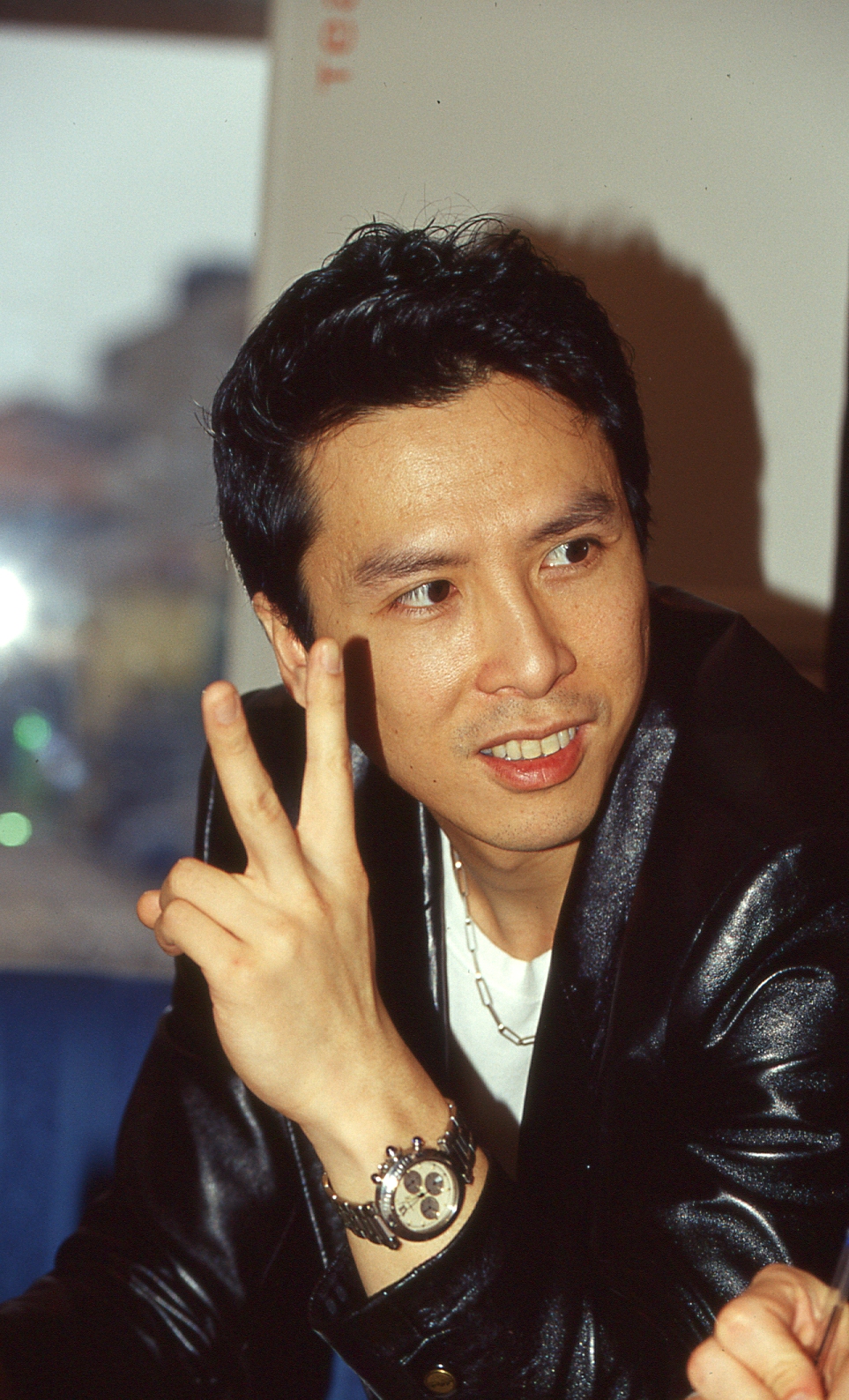The image portrays a young man, possibly in his 20s or 30s, dressed in a black leather jacket over a white shirt, accessorized with a silver watch on his left wrist and a metal-linked chain necklace. He has black, neatly styled hair and tanned skin. He is facing forward but has his head turned to the right, sporting a smile with red lips. His left hand is raised near his face making a "peace" sign with his fingers, and his right elbow is resting on a surface, possibly a table. In the background, a white wall is visible with the shadow of his hair cast upon it, and a blue padded chair appears in the lower left corner. Additionally, there is a light source creating a slight glare on the left side of the picture, and a hand, holding a pen, is seen in the bottom right corner of the image, though the person it belongs to is not visible.